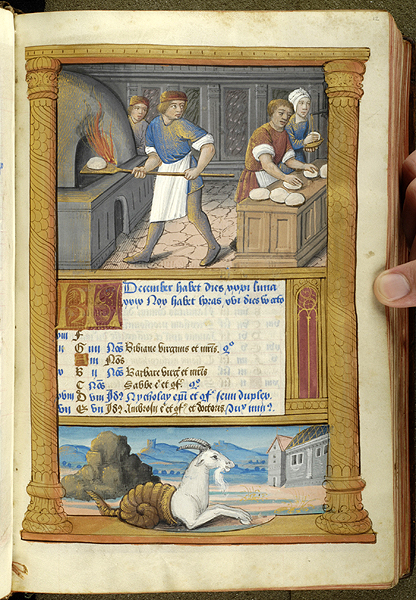The image is a detailed medieval illustration on a page from an old book, held open by a person's hand visible on the right side. The page itself is bordered with a light brown arch that rounds at the top. The upper section of the illustration depicts several people engaged in baking bread. Dominating the left side is a stone oven, with a man wearing a blue shirt, white apron, and brown pants, either placing or removing bread using a peel. On a counter, two individuals, possibly women, are kneading dough, while another person in a blue dress in the background holds a loaf. There are various other loaves on the table in front of them. The middle section contains text in blue and orange fonts, written in an undecipherable language. The bottom illustration features a white goat-like creature with a beard and horns, seemingly emerging from a brown scallop shell or cornucopia. Its hind legs are obscured, possibly hidden inside the shell. In the background, there are buildings and a blue mountain, suggesting a picturesque landscape.